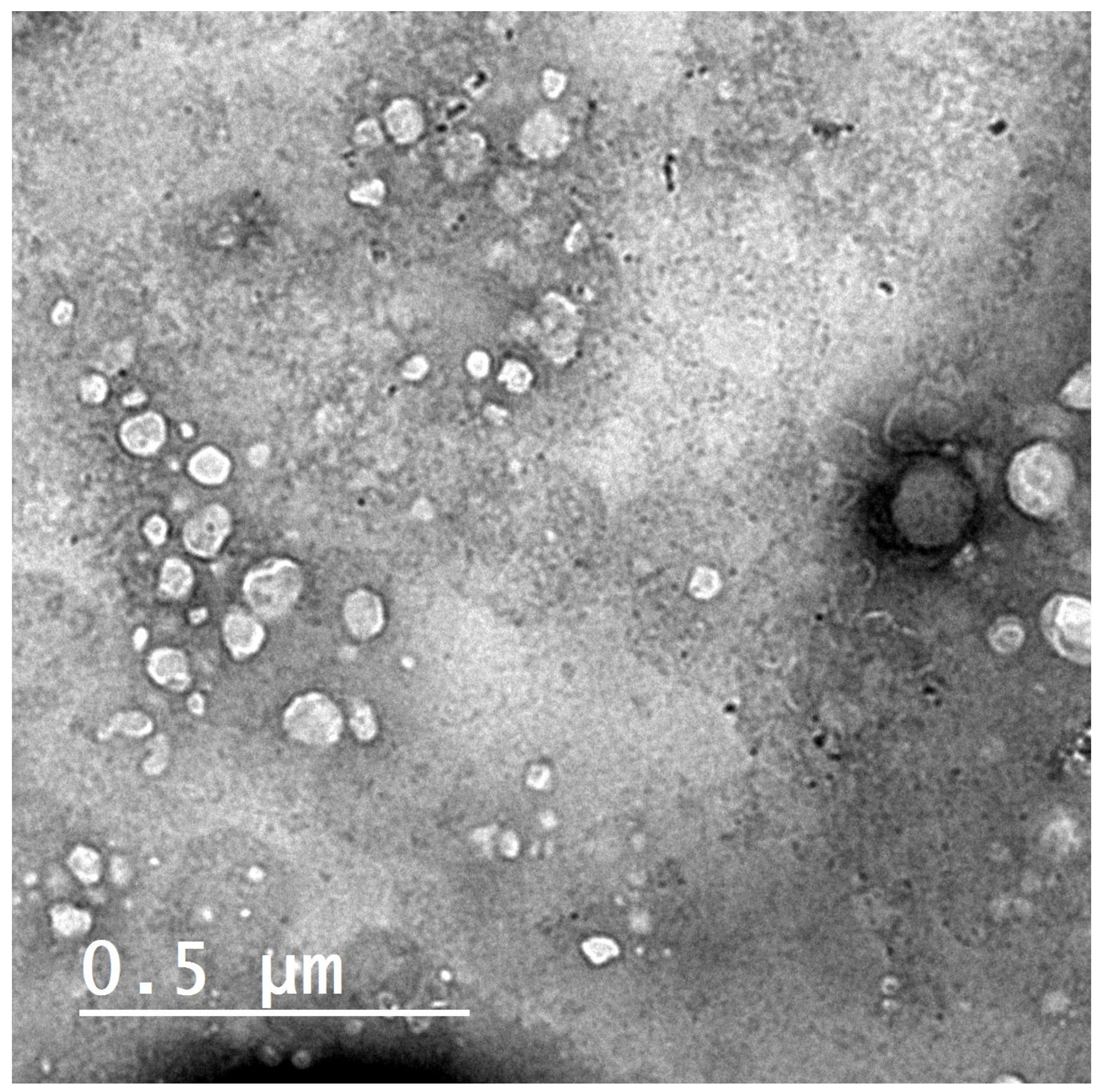This black, gray, and white image appears to be an extremely close-up microscopic view of a sample with a texture similar to pebbled asphalt. In the bottom left corner, a scale bar marked "0.5 µm" (micrometers) provides a measurement reference for the image. The upper left and left areas of the image display several small, white, blob-like circles, which are randomly distributed. On the right side, there's a larger gray circle with a black shadow nearby, and a couple of more substantial white blobs. The image captures fine details that are otherwise indiscernible without magnification, giving it a textured and misshapen appearance, resembling clusters of circular particles.